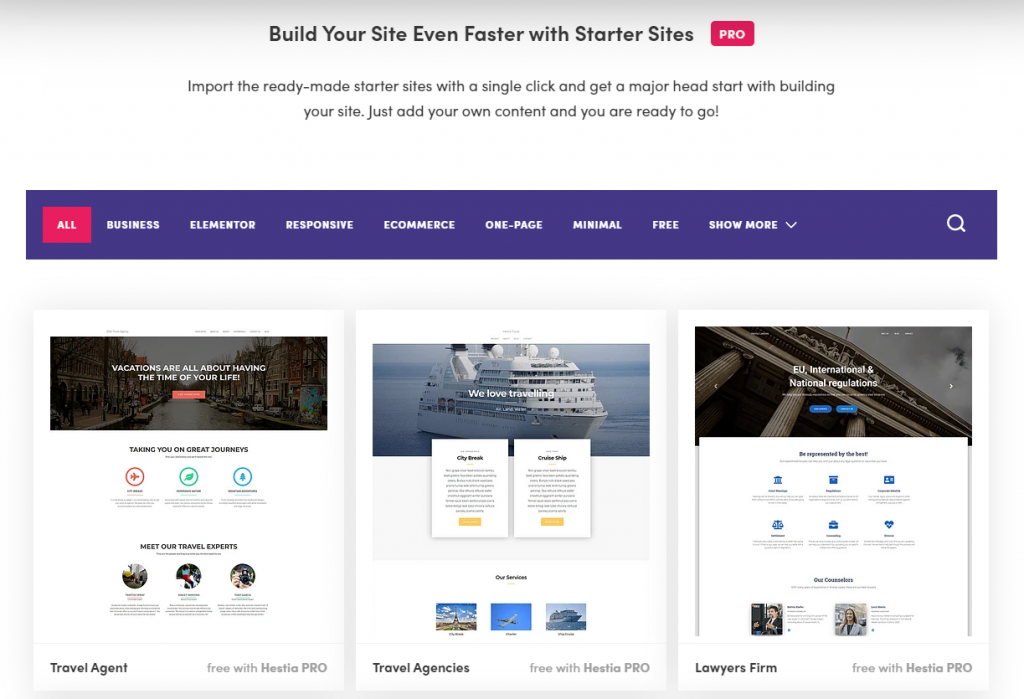This screen capture of a computer or laptop monitor displays a webpage characterized by a deep purple navigation bar at the top. On the far left is a red box with white text reading "ALL," indicating it is selected. Adjacent to this, white text labels continue across the bar, listing categories such as Business, Elementor, Responsive, E-commerce, One-Page, Minimal, Free, and a "Show More" button with a downward-pointing arrow. To the far right, there is a white magnifying glass icon representing a search function.

Below the navigation bar, the content is divided into three main sections. The left section features an evocative image of the Venice canals with a bold white text overlay that reads, "Vacations are all about having the time of your life." Additional text below proclaims, "Taking you on great journeys." This section includes three colorful icons - a red circle with an airplane, a green circle with a leaf, and a blue circle with a bell - and a headline below them that reads, "Meet our travel experts," accompanied by blurry circular images of people. At the bottom left, a tagline states, "Travel agent free with Hestia Pro."

The central section showcases an image of a cruise ship at sea with the heading, "We love traveling." Below this, two boxes are labeled "City Break" and "Cruise Ship." The section also features three icons and corresponding images depicting the Eiffel Tower, an airplane, and a cruise ship, under a header that seems to read "Our Services."

The right section highlights "EU International and National Regulations" with a background image of an ornate coliseum-like building. Despite being blurry, the text below asserts, "Be represented by the best," accompanied by various icons. At the bottom of this section, the text, "Our Counselors," is visible in black, along with blurred images of two individuals, one male and one female. A closing tagline on the bottom left insists, "Lawyers firm free with Hestia Pro."

The webpage appears to offer visually compelling content related to travel, legal services, and various web design categories, unified by the streamlined and professional structure provided by Hestia Pro.